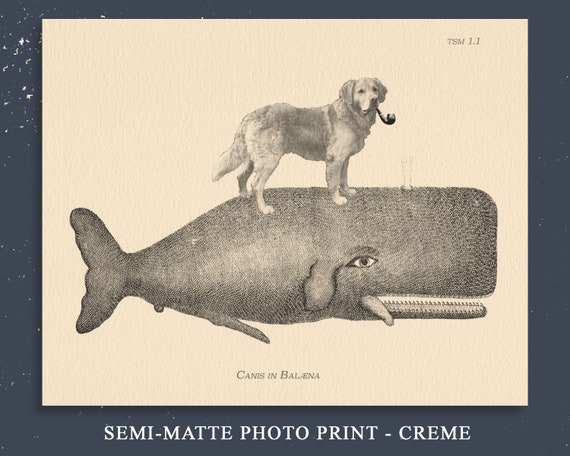This black-and-white image, resembling a semi-matte photo print with a cream background, depicts a surreal and whimsical scene. In the center, a dog, possibly a Golden Retriever or Yellow Lab, is standing on top of a cartoonish whale. The dog has a smoking pipe in its mouth, adding to the oddity of the image. The whale, which has a plume of water spouting from its blowhole, appears to have some sort of object on its head. The scene sits against a faded, beige background, framed with a blue border that features white text reading "semi matte photo print - crème." Below the image, the phrase "canis in ballena" is visible, suggesting an old print style reminiscent of vintage illustrations or maps.